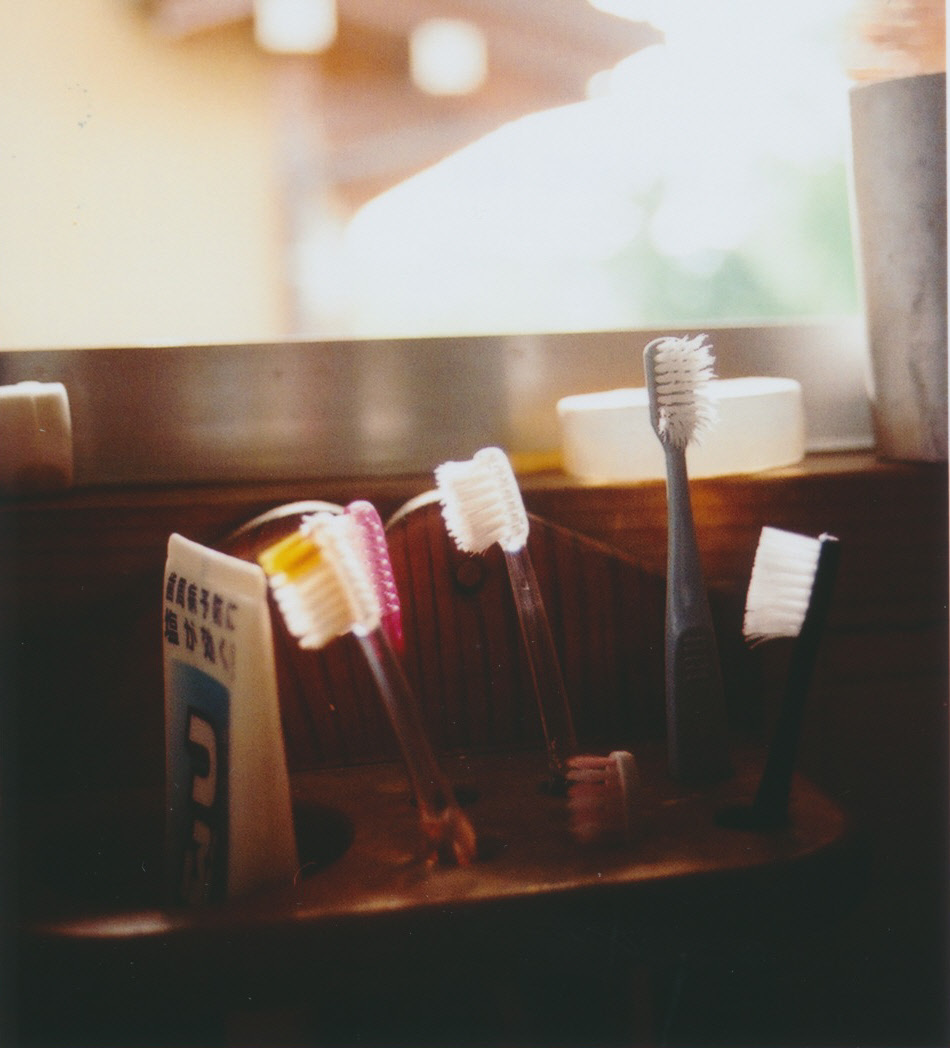The image captures a close-up view of a wooden toothbrush holder containing five toothbrushes with multicolored handles including clear pink, clear dark pink, clear white, gray, and black. Most of the toothbrush bristles are white, except one which has yellow bristles. Accompanying the toothbrushes is a tube of toothpaste featuring blue and white colors with Chinese or Japanese writing on it. The background appears blurry and seems to include a wooden shelf, possibly holding a bar of soap, and a window through which natural light shines, casting a soft glow on the scene. The overall composition lends a serene, yet slightly cluttered ambiance typical of a well-used bathroom.